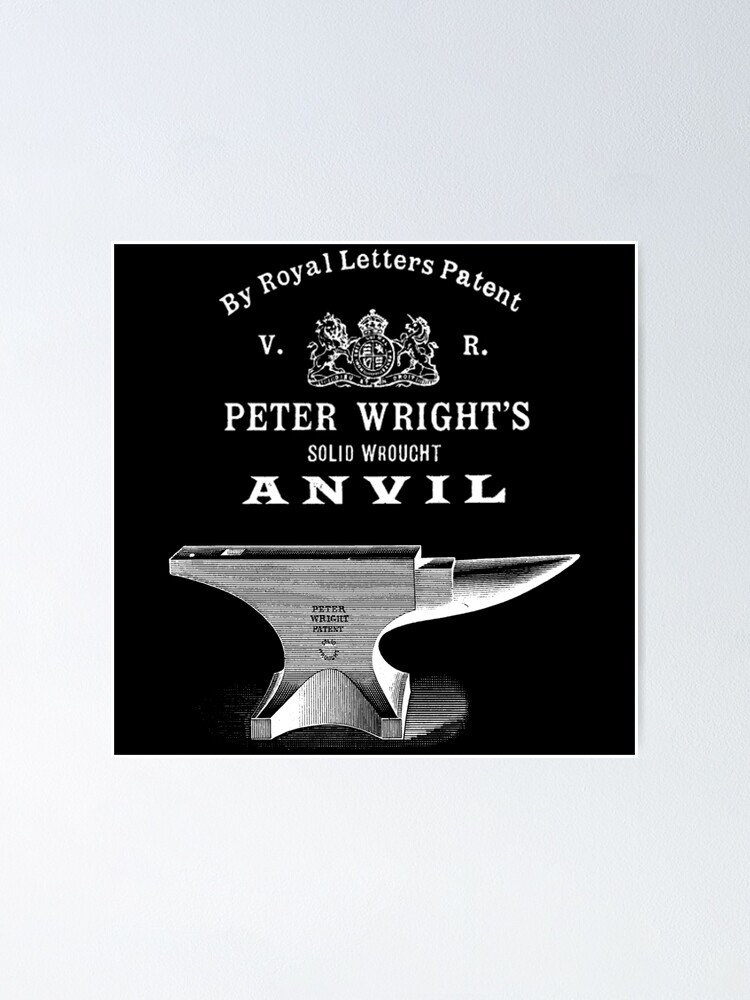The image is a vertically rectangular print measuring approximately six inches in height and four to five inches in width. The background is a light silver-blue tone, with a central black square about two inches by two inches. At the top of the black square, the text arches from the lower left to the upper right, reading "By Royal Letters Patent." Below this text, centered, are the initials "V" and "R" with periods following each letter. Between these initials is a distinguished crest featuring a shield flanked by a lion on the left and a unicorn on the right, topped by a crown. The lower text within the black square reads "Peter Wright's Solid Rot Anvil." Below this inscription is a detailed illustration of a large anvil. The anvil itself is marked "Peter Wright Patent," along with some unreadable circular numbers. The entire design, including the text and graphics, is rendered in gray tones against the stark black background, presumably etched or printed by the brand Etch-It. The image overall showcases the robust and historic nature of Peter Wright's anvil design.